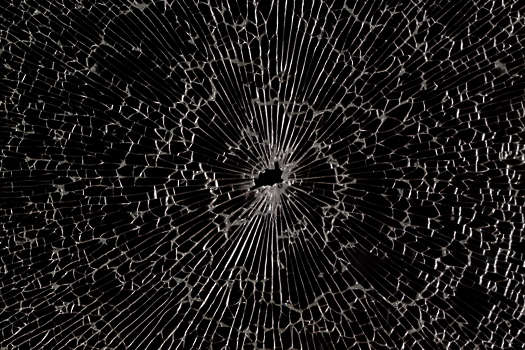This is a detailed close-up photo of a shattered pane of glass against a black background. At the center of the image is a narrow hole, possibly created by a bullet or some other sharp impact, which serves as the focal point. From this central puncture, dozens of straight, white, and gray cracks radiate outward in a spider web-like formation. These cracks extend to the edges of the glass, displaying intricate and varied patterns – some lines are perfectly straight, while others curve and form more abstract, wave-like shapes as they spread outwards. The high contrast between the bright cracks and the uniformly dark background enhances the visual impact of the shattered glass, imbuing the image with an almost surreal, sunburst appearance. Despite the low resolution, the image strikingly captures the delicate and chaotic beauty of the broken glass.